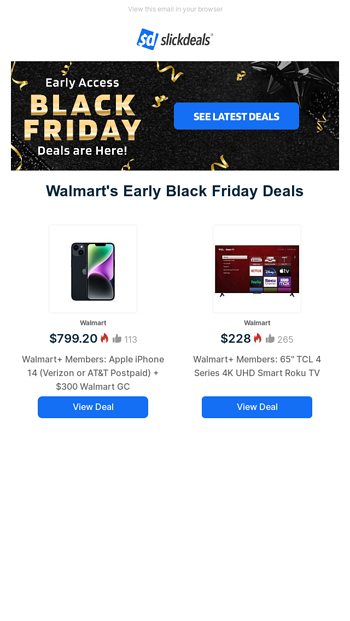This image is a cropped screenshot from the Slick Deals website. At the top center, the Slick Deals logo is prominently displayed. Just below the logo, a large banner exclaims in vibrant, gold lettering, "Black Friday," indicating the presence of early access deals. Centered above "Black Friday" in smaller text, it reads "Early Access." Completing the message, "Deals are Here" is centered below "Black Friday." To the right of this banner, there is a prominent blue button enticing visitors to "See the Latest Deals." The background of the banner is a festive image featuring confetti and bows in black and gold hues.

Beneath the banner, the text "Walmart’s Early Black Friday Deals" appears in bold, dark blue font. To the left under this heading, there's a thumbnail image showcasing the front and back of an iPhone. Accompanying the thumbnail is the price of the iPhone, highlighted alongside a brief description. At the bottom of this section, centered text prompts users to "View Deal."

On the right side, a similar layout features a TCL 4K UHD Smart Roku TV. Its price and description are displayed in the same format as the iPhone deal. Notably, a small fire icon appears next to each price, indicating a hot deal.